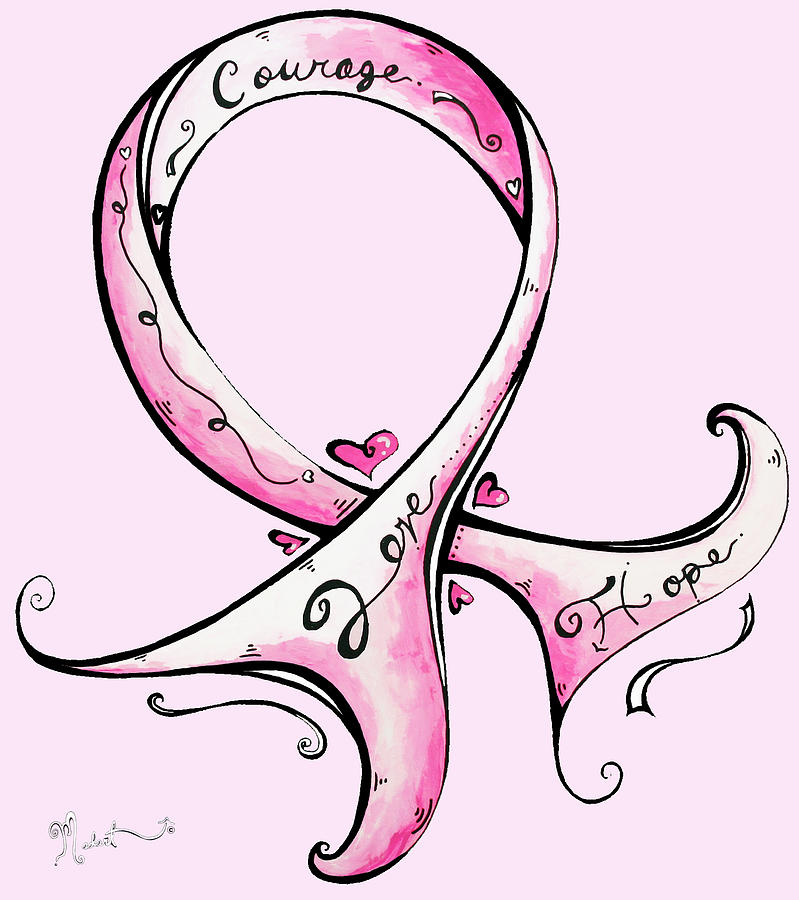This hand-drawn computer-animated image or tattoo-like illustration features a prominent circular ribbon often associated with various causes, colored in light pink, dark pink, and white hues. The ribbon displays the word "COURAGE" at the top in black cursive letters and the word "LOVE" in the lower part of the loop, also in black cursive. To the right edge of the ribbon is the word "HOPE" in bold cursive with a capitalized "H." The ribbon is accented with four hearts: one large heart positioned centrally within the ribbon and three smaller hearts surrounding its edges. There are also swirling decorative lines and design elements throughout the ribbon. The entire drawing is outlined in black, and an artist's signature appears at the bottom left in cursive white writing, though it is not legible.